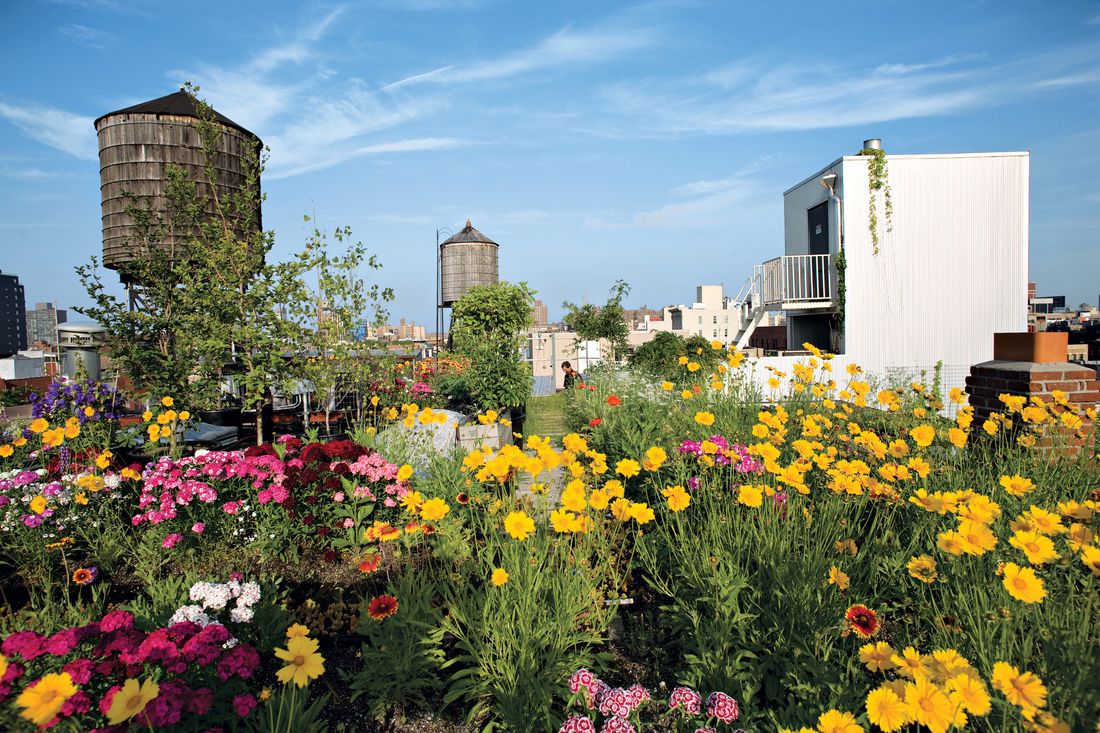The image features a vibrant rooftop garden brimming with blooming flowers of various colors and types. The bottom half of the photograph is adorned with a dazzling array of yellow flowers that resemble dandelions or daisies, each with long stems, accompanied by a mix of beautiful purple, dark pink, pink, and red blossoms, along with some soothing greenery. Prominently, there are two elevated water towers visible to the left, providing a sense of the rooftop's height. Adding to the scene's charm is a small white building fitted with stairs, presumably the access point to the rooftop. In the distance, a person, whose gender is hard to discern, tends to the flourishing garden, further highlighting the space's serene and meticulously cared-for nature. The flowers, diverse in size and shape, create a picturesque and vibrant setting against the urban backdrop.